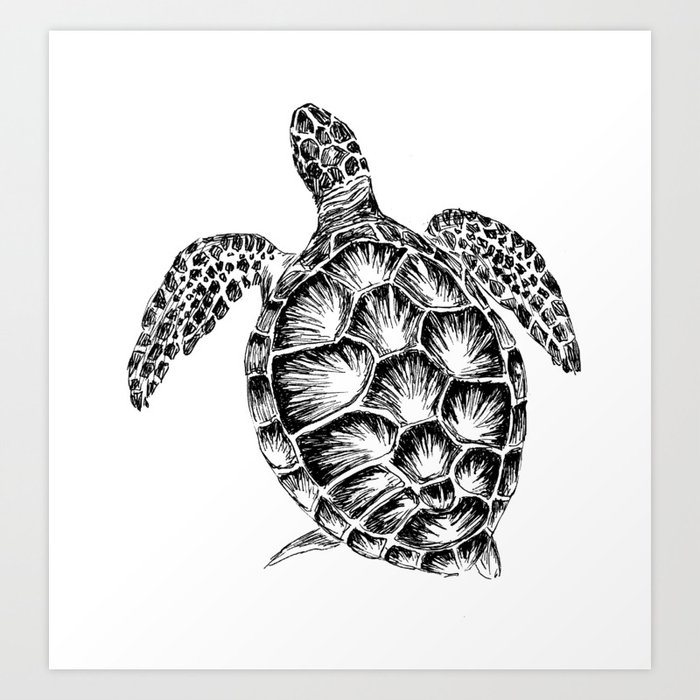This is a highly detailed, black and white, hand-drawn image of a giant sea turtle viewed from a top-down perspective, either hanging on a wall or laid flat on a table. The sea turtle's distinct fin-shaped limbs, head, and back fins—suitable for swimming—are all extended and visible, with no part retracted into its shell, confirming it as a sea turtle. The drawing appears to be done with pencil or black ink, emphasizing intricate shell patterns that resemble fire-like designs within each segment of the shell. The turtle, positioned centrally in an otherwise plain white background, features meticulously drawn flapper arms adorned with black dots and similar designs as seen on the shell and head. The turtle’s head is oriented towards the top of the image, enhancing the bird's eye view effect. The artwork focuses solely on the turtle, with no eyes, additional identifying features, or text present in the image.